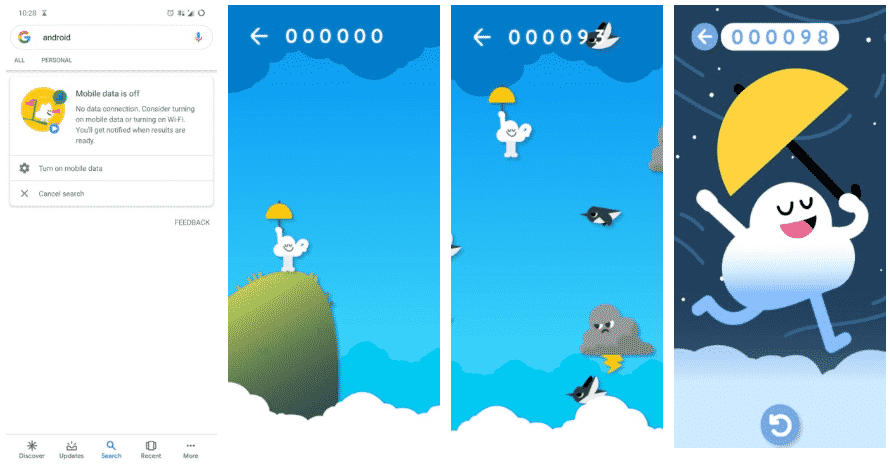This image is a detailed screenshot from a Google Play Store page, likely captured on a tablet given the screen dimensions. On the left-hand side, the white background contains status icons in black at the top left, displaying the time as 10:29 without specifying AM or PM. Alongside, there is a grey hourglass, followed by a clock and a star-like symbol, indicating various statuses. A nearly full cell phone signal icon sits alongside another grey circle. Next is a circular icon featuring the Google logo in red, yellow, green, and blue, labeled "Android" in black. Adjacent, a blue pill-shaped icon is underlined by red and blue lines.

Further down, a new section begins, marked by a rectangle containing an orange circle with a red flag on a green pole. Inside this section, a white cloud-like figure with black eyes and mouth holds a red bullhorn. Below is a blue circle with a white right-pointing arrow, followed by bold black text stating "Mobile data is off." Regular black text underneath explains, "No data connection. Consider turning on mobile data or turning on Wi-Fi. You will get notified when results are ready." A dark black gear icon appears within a thin-bordered rectangle, accompanied by light black text reading "Turn on mobile data." A dark grey "X" and the words "Cancel search" appear next, followed by a "Feedback" link on the right.

In the central area, the background features dark blue hues with lighter blue cloud-like forms resembling storm clouds. The first light-green to dark-green gradient rectangle depicts a character standing on a bean-shaped grassy ledge, surrounded by white clouds. This character, a cloud-like figure with a yellow umbrella and mid-grey feet, has black eyes and a black mouth. On the adjacent right side, this figure floats with black and white birds beside an ominous dark grey and mid-grey cloud, characterized by black eyes, a black mouth, and a yellow lightning bolt. Another area contains a bold white arrow with "0000009379" and a black and white bird.

On the right-hand segment, a dark blue background with light blue swirls simulates wind. Here, the close-up cloud character, with a hot pink tongue, sings with closed black eyes while holding a yellow umbrella. At the top of this section, a blue circle with a bold white arrow and adjacent blue numeric figures "498" immediately catch the eye. Beneath this, a blue and white cloud, paired with a blue circle displaying a white refresh symbol, concludes the details.